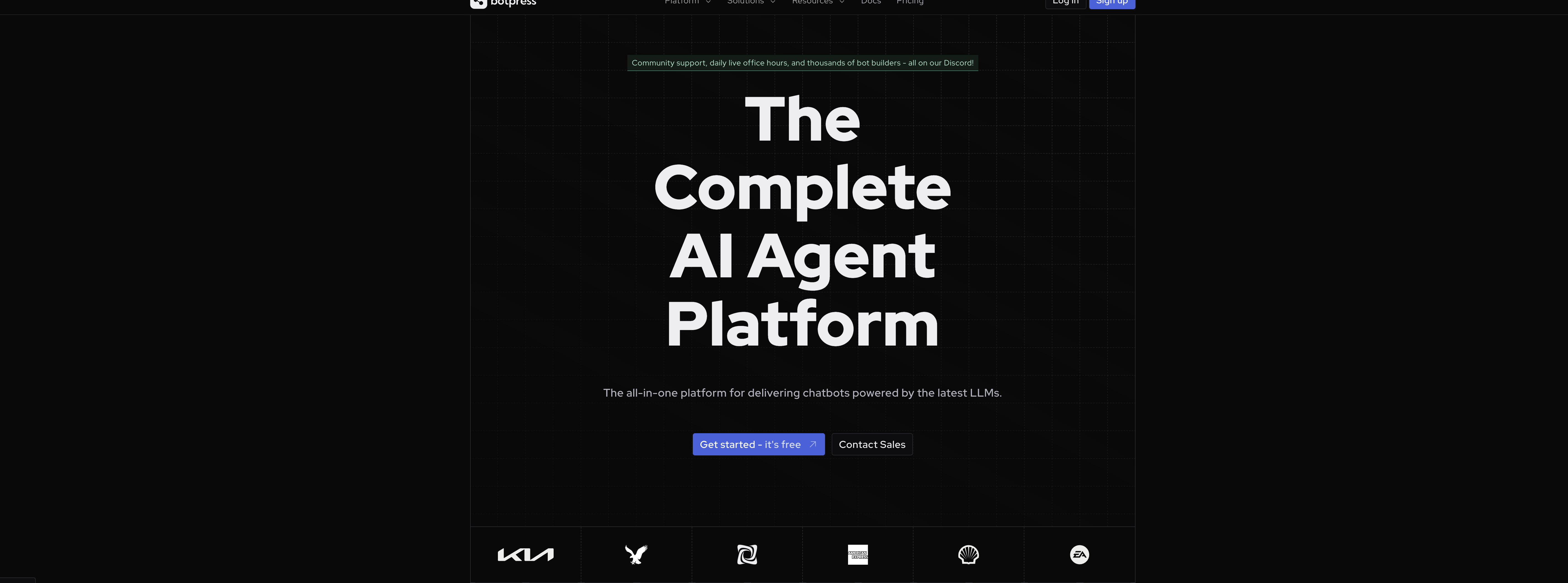The image displays a screenshot of an error or verification page from Cloudflare. The background is predominantly white, creating a clean and uncluttered look. At the top left corner, there is a URL: "botpress.com." Beneath this, it states, "Checking if the site connection is secure."

A gray box is prominently featured in the center. On the left side of the box, the word "Verifying" is displayed alongside a green loading icon, indicating that a check is in progress. To the right, there's the word "Cloudflare" accompanied by Cloudflare's distinctive orange cloud logo.

Further down, a message reads, "botpress.com needs to review the security of your connection before proceeding," signaling that some security checks are being performed. At the bottom of the page, there is a clickable section labeled "Why am I seeing this page?"

The footer of the page contains the text, "Performance & security by Cloudflare," with the word "Cloudflare" appearing as a blue hyperlink. Directly above this, an ID number is displayed, likely for reference purposes.